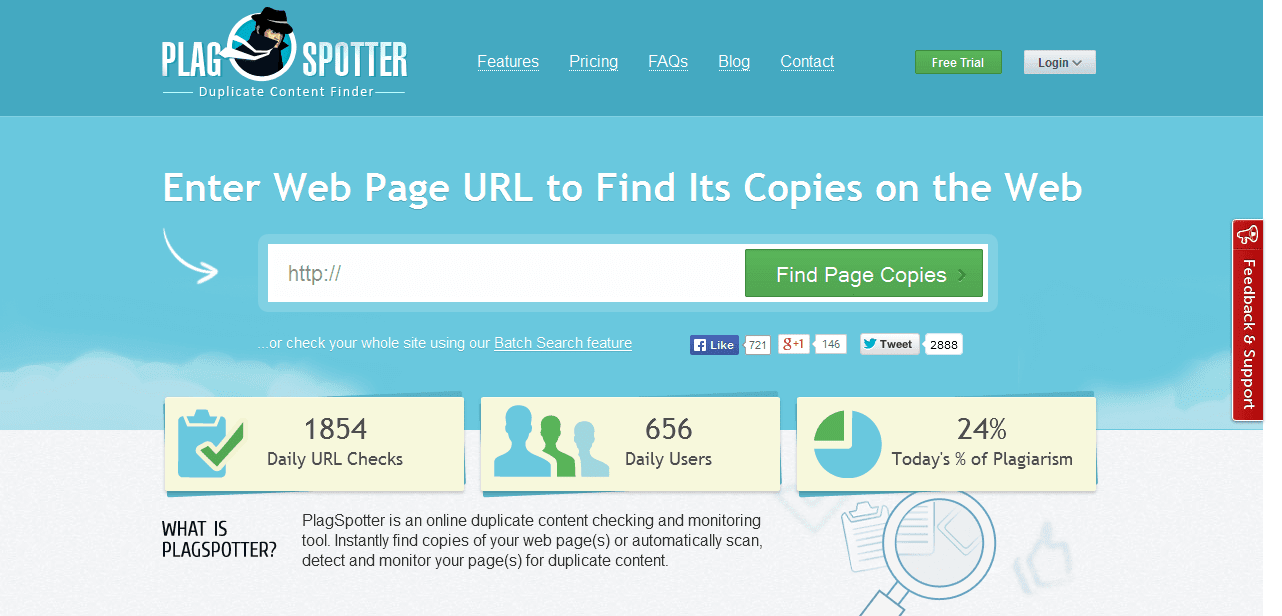The interface displays the "Plagg Spotter" duplicate content finder, prominently in white text. Positioned between the words "Plagg" and "Spotter", there is a black icon featuring a man in a trench coat, a black hat, and a white tie flowing behind him, all set against a dark turquoise band. Centrally aligned on the band are navigation options: "Features," "Pricing," "FAQs," "Blog," and "Contact," all underlined in white. To the right, there is a green button with white text that says "Free Trial," followed by a gray button labeled "Log In," which includes a pull-down menu below it.

The background of the page is a lighter turquoise or teal color. Below the band, white text prompts users to "Enter web page URL to find its copies on the web," next to an arrow pointing towards a data input field pre-filled with "http://," ready for user input. Adjacent to the field, a green button with white text says "Find Page Copies."

Further down, the text suggests an alternate option to "...or check your whole site using our batch search feature," with "batch search feature" underlined. There is also a set of social media buttons indicating popularity metrics: "Like on Facebook" showing 721 likes, "Google Plus" with 146 endorsements, and "Twitter," showcasing 2,888 tweets.